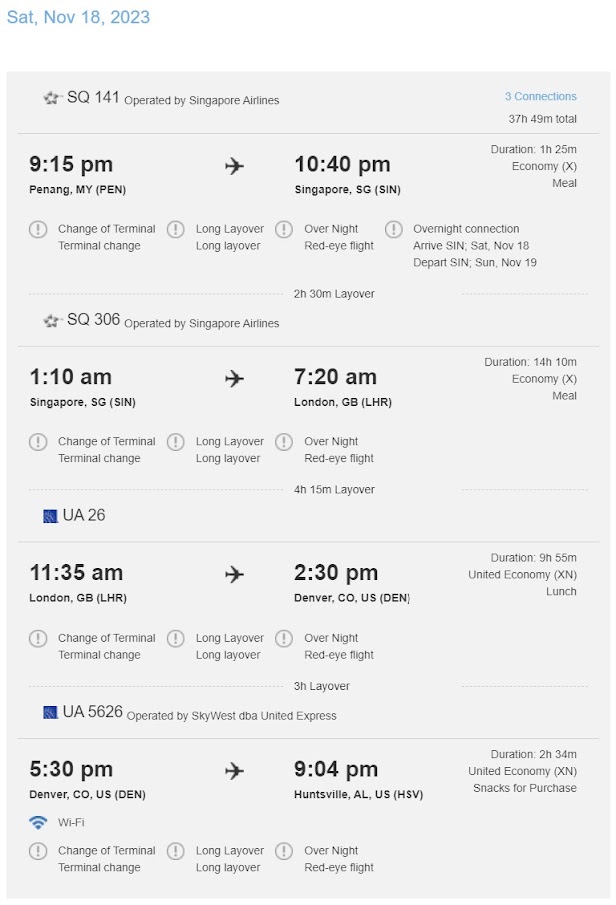The image depicts a flight booking page with multiple details about the journey. In the upper left corner, there is the date "Saturday, November 18, 2023," printed in blue font on a white background. The main page features a gray background with black and gray text.

In the top left of the main section, the flight information shows "SQ1," indicating a flight operated by Singapore Airlines. To the right, in blue text, it mentions "3 connections" and a total travel time of "37 hours 49 minutes."

Further down, it states the departure time as "9:15 PM" from Penang, Malaysia (PEN), and the arrival time as "10:40 PM" in Singapore (SIN). The duration of this leg is "1 hour 25 minutes." The booking class is "Economy X," and it includes a meal.

Below this section, there is a notice about a terminal change and an overnight red-eye flight. The connection arrives on Saturday, November 18, and departs on Sunday, November 19. A line separates the information segments, below which it indicates a "2 hour 30 minute layover."

Continuing, it lists another flight "SQ306," also operated by Singapore Airlines, with a departure time of "1:10 AM."